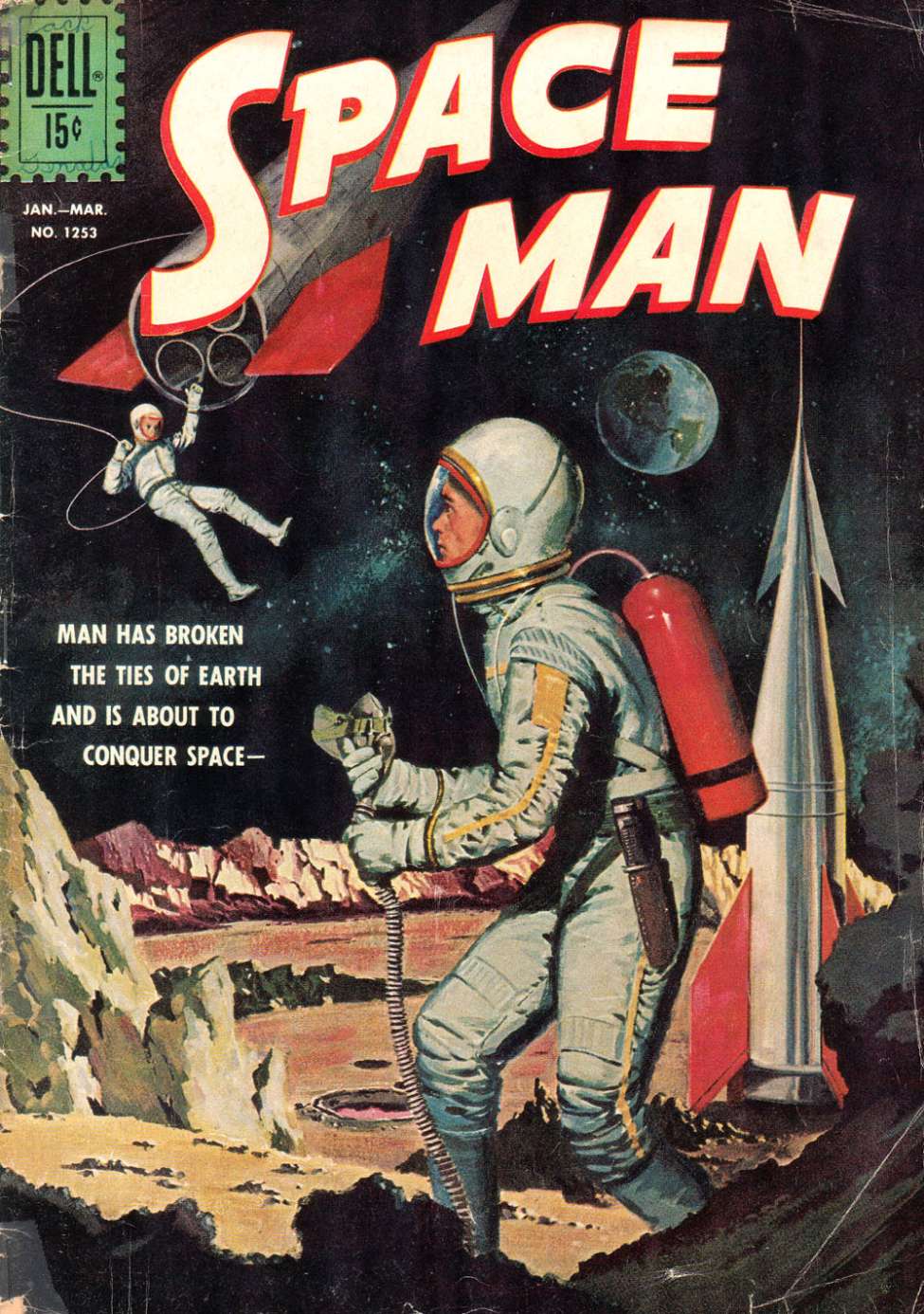The image appears to be the cover of an old-school comic book or magazine. In the top left is a small green, perforated rectangle resembling a stamp, with bold black text in all caps reading "DELL" underlined, followed by "15¢." Beneath this in white text, it reads "JAN-MAR NO 1253," indicating the publication date and issue number. 

The title of the publication, "SPACEMAN," is prominently displayed in large white letters with a red three-dimensional outline, with "SPACE" positioned above the word "MAN." 

The main illustration features two astronauts in a space setting. In the foreground is a male astronaut, standing amidst the rocky terrain of a reddish-brown and orange-yellow planet, possibly Mars. He wears a white spacesuit with yellow stripes along the arms and legs, and dons a helmet with a glass visor. His equipment includes a brown-sheathed knife at his hip and a red oxygen tank with a metallic tube connected to his back. He also holds a corrugated tube or pipe.

In the background, floating in space attached to a cord extending from a rocket, is a second astronaut. This astronaut, potentially a woman, appears to be waving, with an arm raised. The rocket, partially obscured by the title "SPACEMAN," features red fins and multiple booster rockets.

Below the word "MAN" is the depiction of a planet, likely Earth, shrouded partly in shadow with visible dark blue, green, and black land masses. The planet in the scene is characterized by jagged, dark rocky formations at the front, with vertical rocks and craters enhancing the rugged landscape. 

Overall, the illustration is vibrant and detailed, with a dark outer space background highlighting the astronauts' white suits and the colorful planetary surface.